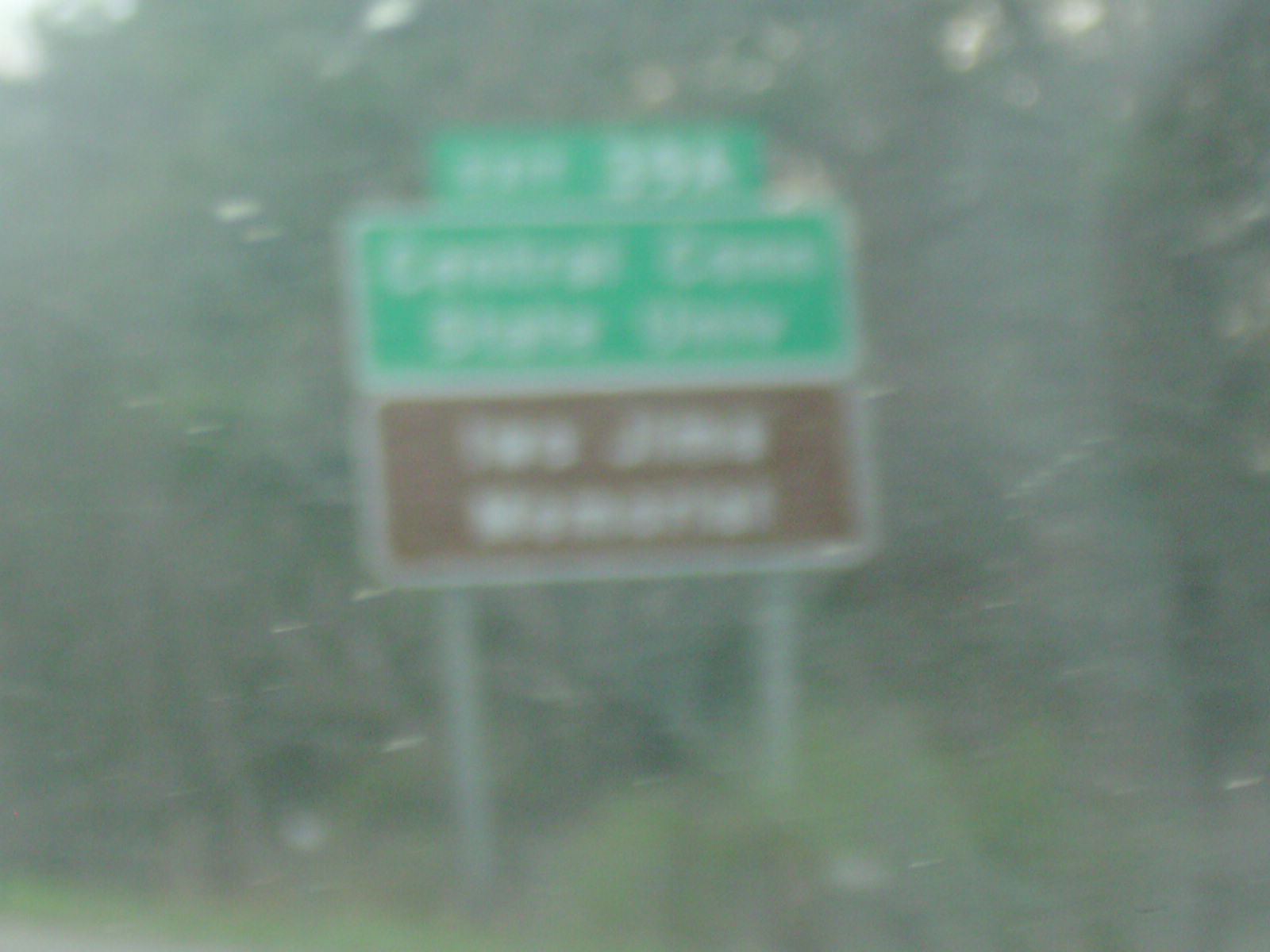This photograph, taken from the interior of a moving vehicle, captures a roadside sign in a rather obscured manner. The view through the car window is compromised by multiple factors: the glass is notably dirty with light white and tan dirt marks, the image appears blurred, likely due to both the motion of the car and the condition of the window. The sign itself consists of three components: at the top, a smaller, narrow rectangle with white lettering indicating the upcoming exit; below that, a larger green rectangle with additional white text; and at the bottom, a brown rectangle also featuring white lettering. The background scenery includes a patch of bright green grass and some brown trees adorned with dark green leaves. The overall lack of clarity makes reading the specific details on the sign difficult.